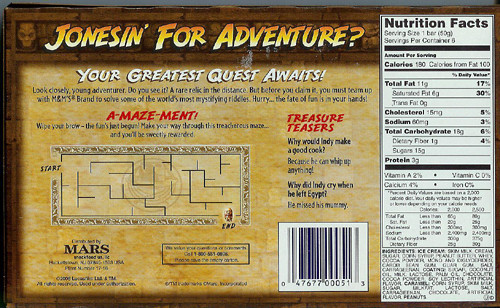Detailed Caption:

This is an image of the back of a food product box. At the top, bold yellow text reads, "Be jonesing for adventure?" To the right of this text, there is a white nutritional facts table with black lettering, detailing the product's nutritional information. Below and to the left of the nutritional facts, large white text proclaims, "Your greatest quest awaits." The central section of the box showcases a maze, inviting interaction. Directly to the right of the maze, in the middle of the box, sits a barcode.